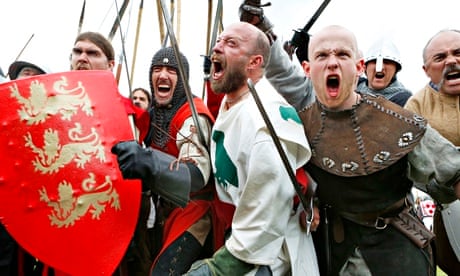In this outdoor medieval reenactment scene, a group of fervent warriors, some clad in English knight armor, are captured in mid-shout beneath a lighter, overcast sky. On the far left, a standout figure wields a conspicuous red shield adorned with three golden lion designs. Central to the image is a man draped in a white robe marked with green, possibly featuring a bird motif, reminiscent of a monk's attire. Another notable participant, with a shaved head, dons a brown uniform. Further back, a figure in a metal helmet equipped with a nose protector is seen with a metal shirt hanging down the middle. Many of the warriors brandish swords, with some wearing chainmail, robes, and large gloves. Beards and mustaches are common among them as they all face the camera, contributing to the intense, dramatic energy of the reenactment.